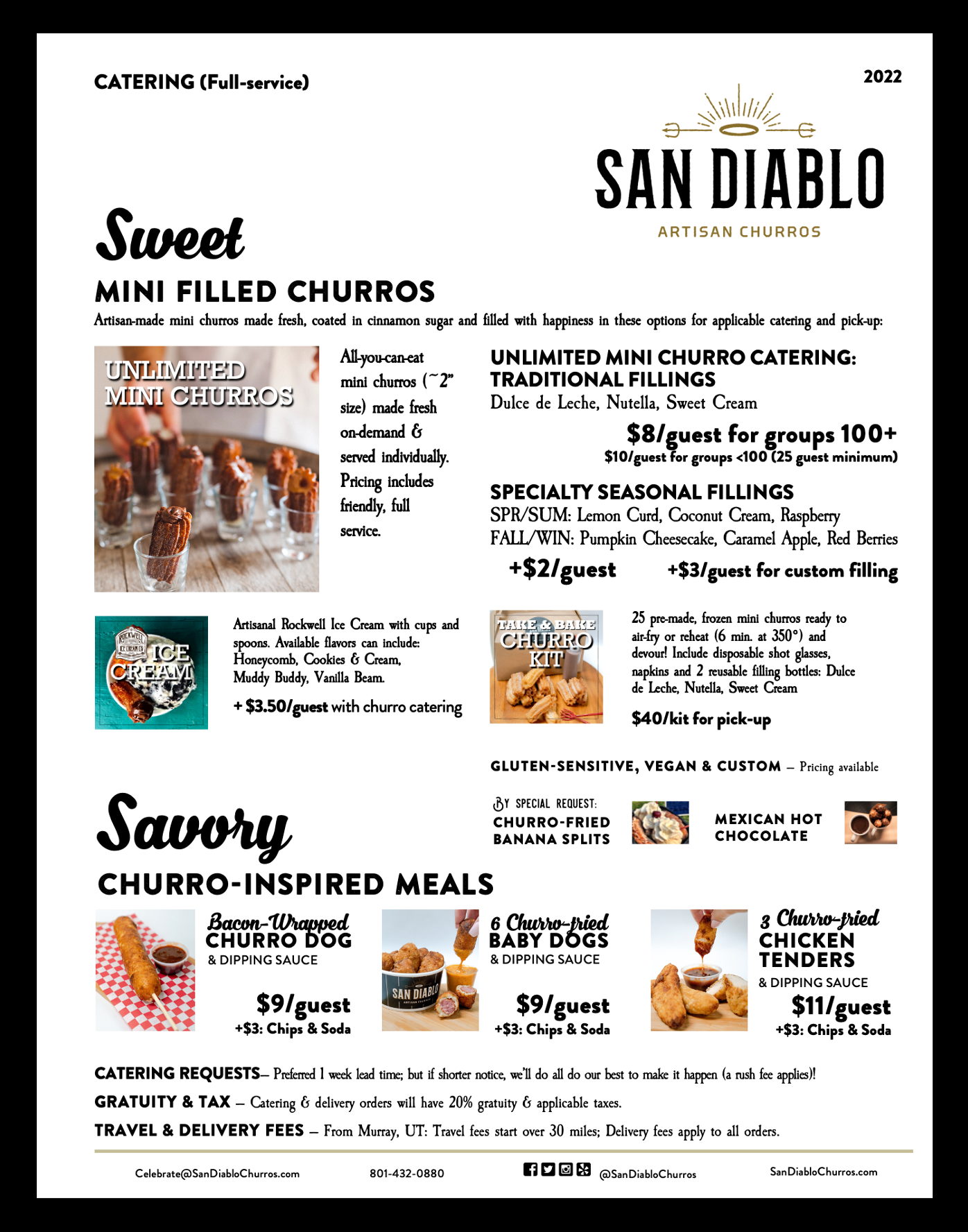The image displays a rectangular catering menu for "San Diablo Artisan Churros," framed by a thick black border on a white background. The top left corner of the menu reads "Catering (Full Service)," while the top right corner displays "2022." Adjacent is a golden logo featuring two pitchforks with a radiating halo, under which "San Diablo" appears in black capital letters, followed by "Artisan Churros" in gold text.

The menu is divided into two main sections, marked by bold, black cursive text: "Sweet" and "Savory." Under the Sweet section, various items are listed starting with "Mini Filled Churros," described as artisan-made, mini churros coated in cinnamon sugar and filled with various flavors. Options include unlimited mini churros for catering priced at $8 per guest for groups of 100 or more, with additional options for specialty seasonal fillings such as lemon curd and pumpkin cheesecake. Also featured are churros served with ice cream at $3.50 per guest, and take-and-bake churro kits available for pickup at $40.

The Savory section highlights "Churro Inspired Meals," listing items like "Bacon Wrapped Churro Dogs" and "Churro Fried Chicken Tenders," with corresponding pricing per guest. 

At the bottom of the menu, there's detailed information on catering requests, gratuity, tax, travel, and delivery fees, including specifics like a 20% gratuity and travel fees starting from Murray, UT for distances over 30 miles. The footer also includes contact information, URLs, and social media handles for further inquiries.